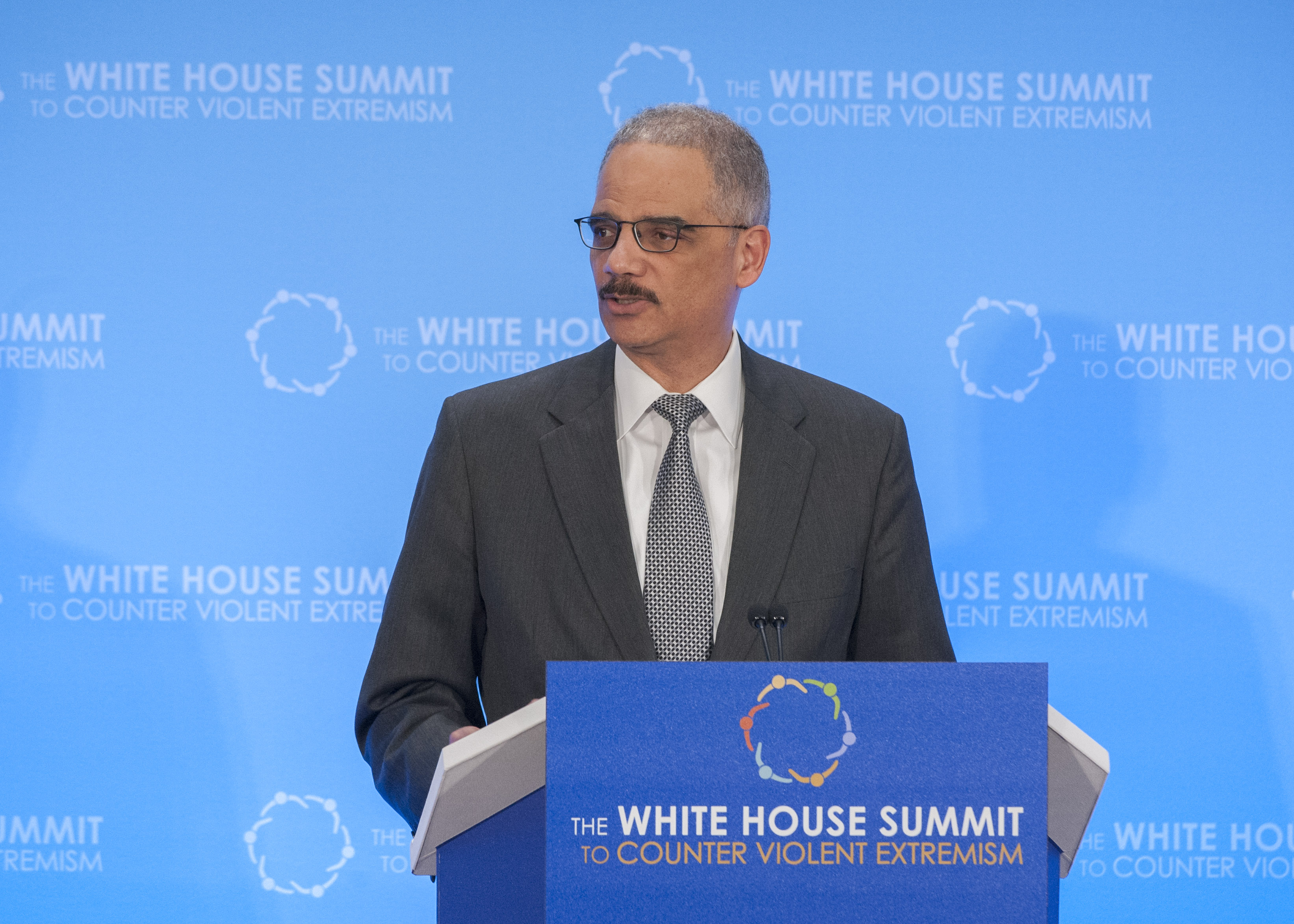In this image, a distinguished man, who appears to be Eric Holder from the Obama administration, stands at the center wearing a dark gray suit jacket with a white collared shirt and a gray-and-white tie. His short, graying hair, black eyeglasses, and mustache accentuate his tall, slim figure. He has caramel-colored skin. Holder is positioned behind a blue podium that bears the text "The White House Summit to Counter Violent Extremism," accompanied by a multicolored logo and orange and white text. The podium also holds stacks of white papers on either side and is equipped with two small microphones. The backdrop features a large, light blue poster displaying the same summit text, creating a cohesive setting that highlights the importance of the event.